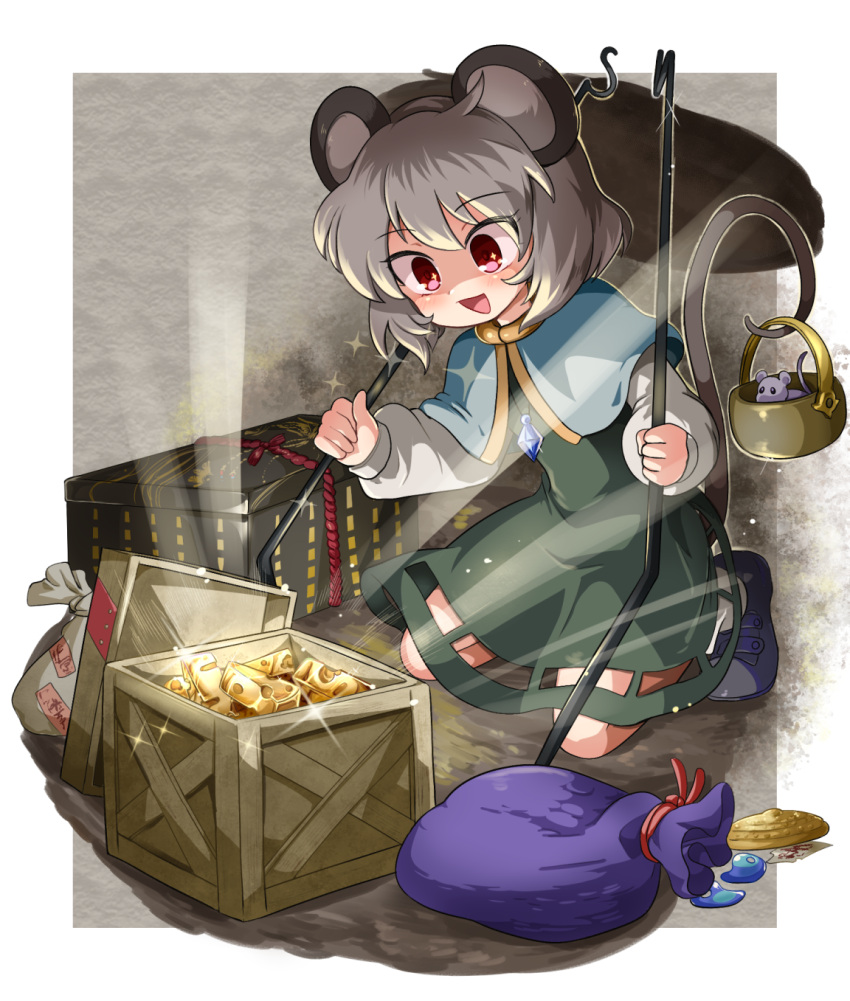This captivating anime-style illustration depicts a young mouse-girl with large, expressive eyes and short, light gray hair topped with big, mouse-like ears. She is dressed in a dark green dress and a light blue cape with gold trim, complemented by a dark blue amulet at her neck. Kneeling on the floor, she is holding a bar with a crimp on the end over her shoulder and a crowbar in her left hand, indicating her role as a treasure seeker. Her mouse tail, notably, is wrapped around a small kettle holding a tiny mouse. 

The focal point of her gaze is an open wooden chest brimming with shiny, glimmering gold that illuminates her and the surrounding scene. Next to the chest is a purple bag tied with red string, resembling a small Santa sack, hinting at another treasure. In the background, a gray, textured setting adds to the mystical atmosphere, with another package tied shut sitting nearby. The mouse-girl's expression is one of amazement and joy, reveling in her newfound trove of glittering treasures.